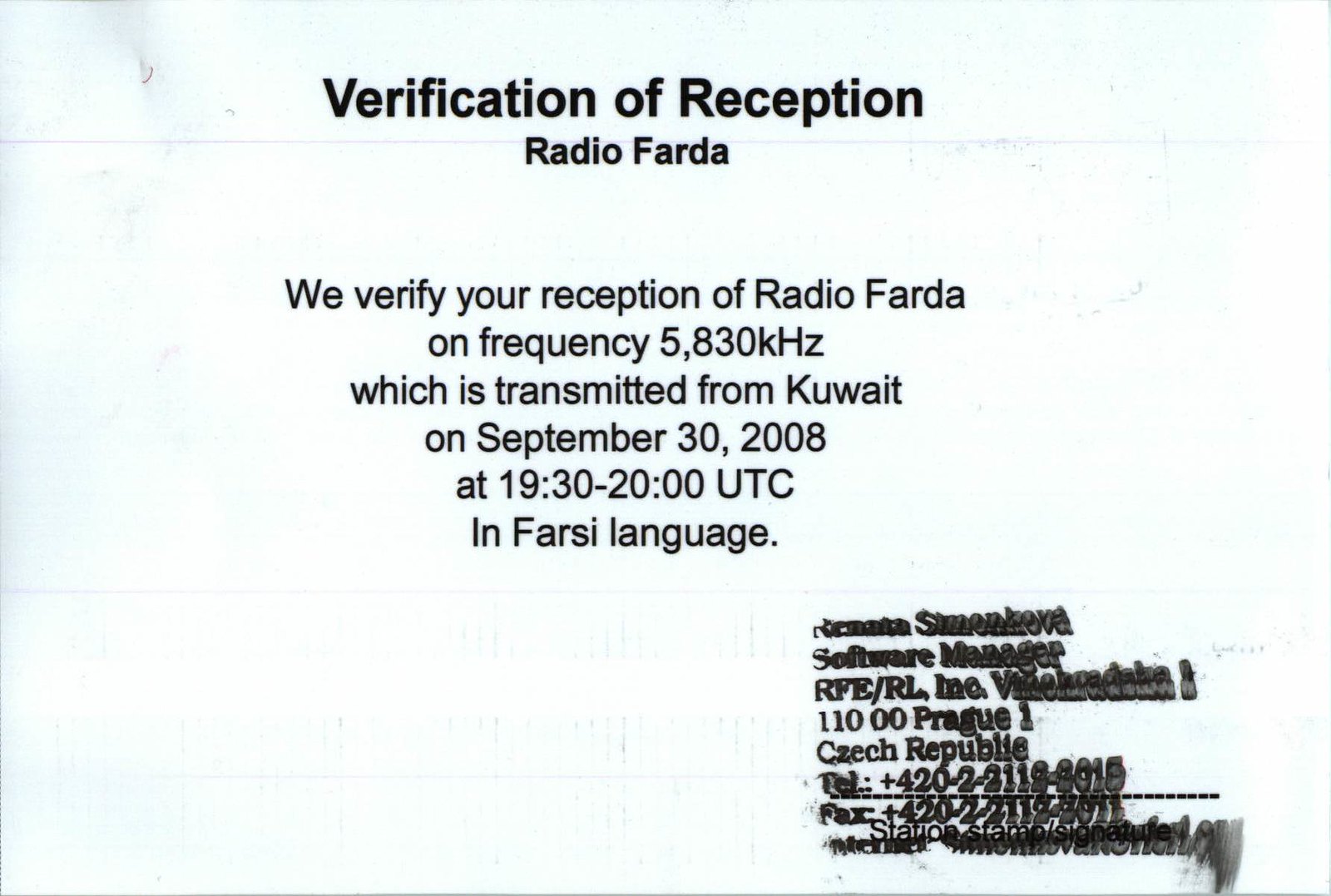The image features a verification of reception from Radio Farda, displayed in bold Arial font on a white background. At the top, it prominently states "Verification of Reception, Radio Farda" in bold type. Below this, the text verifies the reception of Radio Farda on the frequency 5,830 kilohertz, transmitted from Kuwait on September 30, 2008, at 19:30-20:00 UTC, in the Farsi language. On the lower right of the image is a stamp that is somewhat smudged, making the details blurry. It reads "Renata Sinonkova, Software Manager, RFE/RL Inc., 11000 Prague 1, Czech Republic," and contains additional contact details. A dotted line runs along the bottom part of the image.